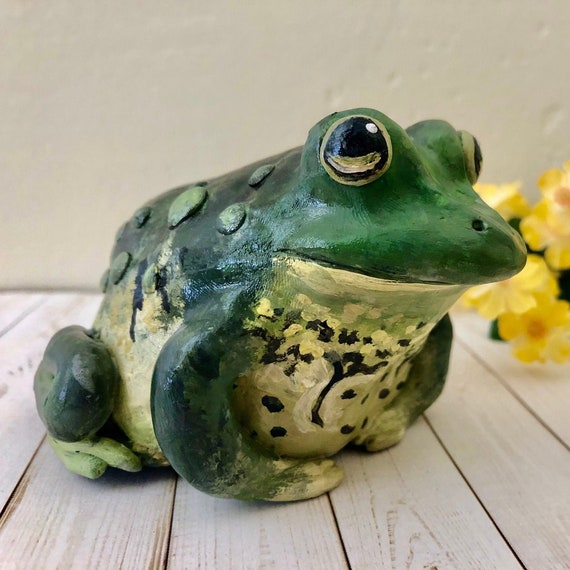The image features a detailed porcelain frog statue, painted predominantly green with some variations in shade, with the front being a lighter green and the back a darker green. The frog is positioned on a wood-grained floor, or perhaps a deck or table, against a cream-colored wall. The statue displays intricate details such as black eyes with hints of yellow around them, and a mixture of green, yellow, and black coloring on its underbelly and chest. The frog's arms and legs are green, with one leg bent under its body. Its skin features small warts or bumps, adding to the lifelike appearance. To the right side of the frog, vibrant yellow flowers provide a contrasting and colorful backdrop. The frog is facing to its right, displaying a nuanced mix of colors and textures that lend realism to the artwork.